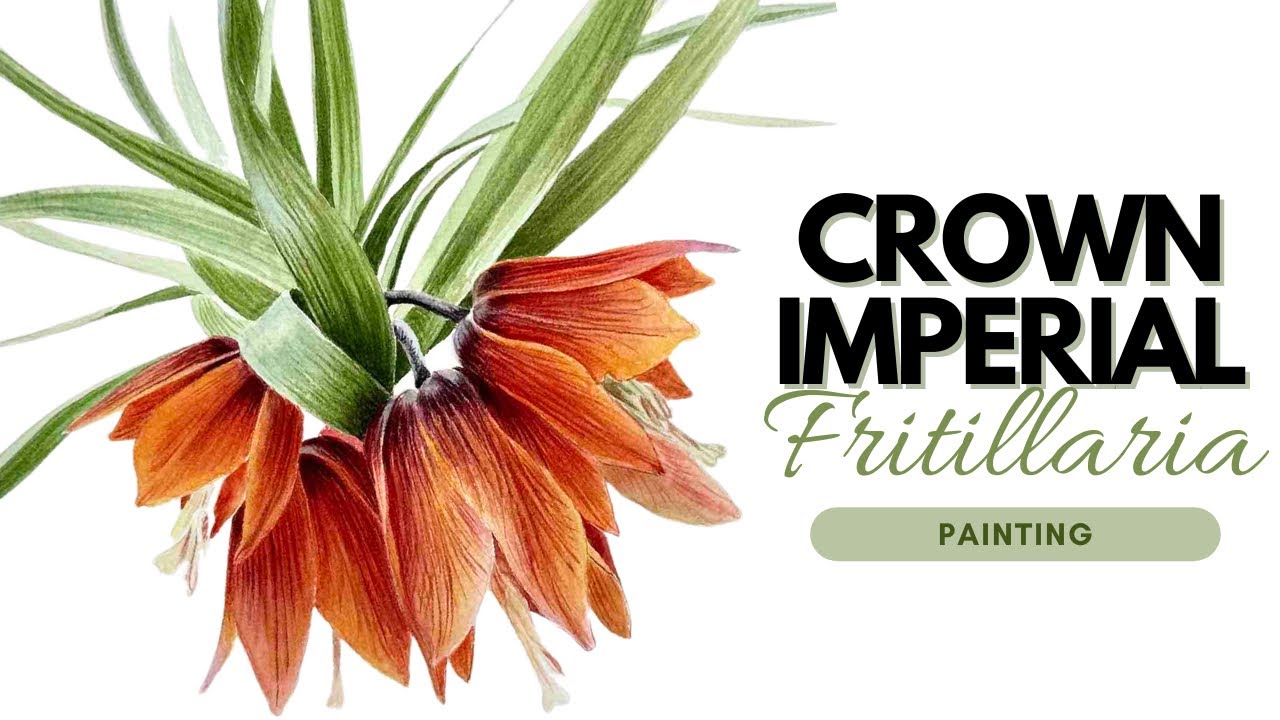The image appears to be an advertisement or poster for a painting titled "Crown Imperial Fritillaria." On the right side, the title is displayed. "Crown Imperial" is written in strong, dark brown or black print, while "Fritillaria" is in a lighter green cursive font. Below these titles, in a slightly darker green, is the word "painting," encased in an oval green box, indicating a clickable element, possibly suggesting a website interface.

On the left side of the image, there is a detailed illustration of a Crown Imperial Fritillaria plant. The plant features long, dark green leaves and four dingy-looking, orangish-reddish flowers. The flowers dangle from the stems with visible white stamens, capturing the essence of this beautiful, flowering plant. The background is predominantly white, creating a clean and minimalist look that emphasizes the vibrant colors of the plant and the elegant typography of the text.